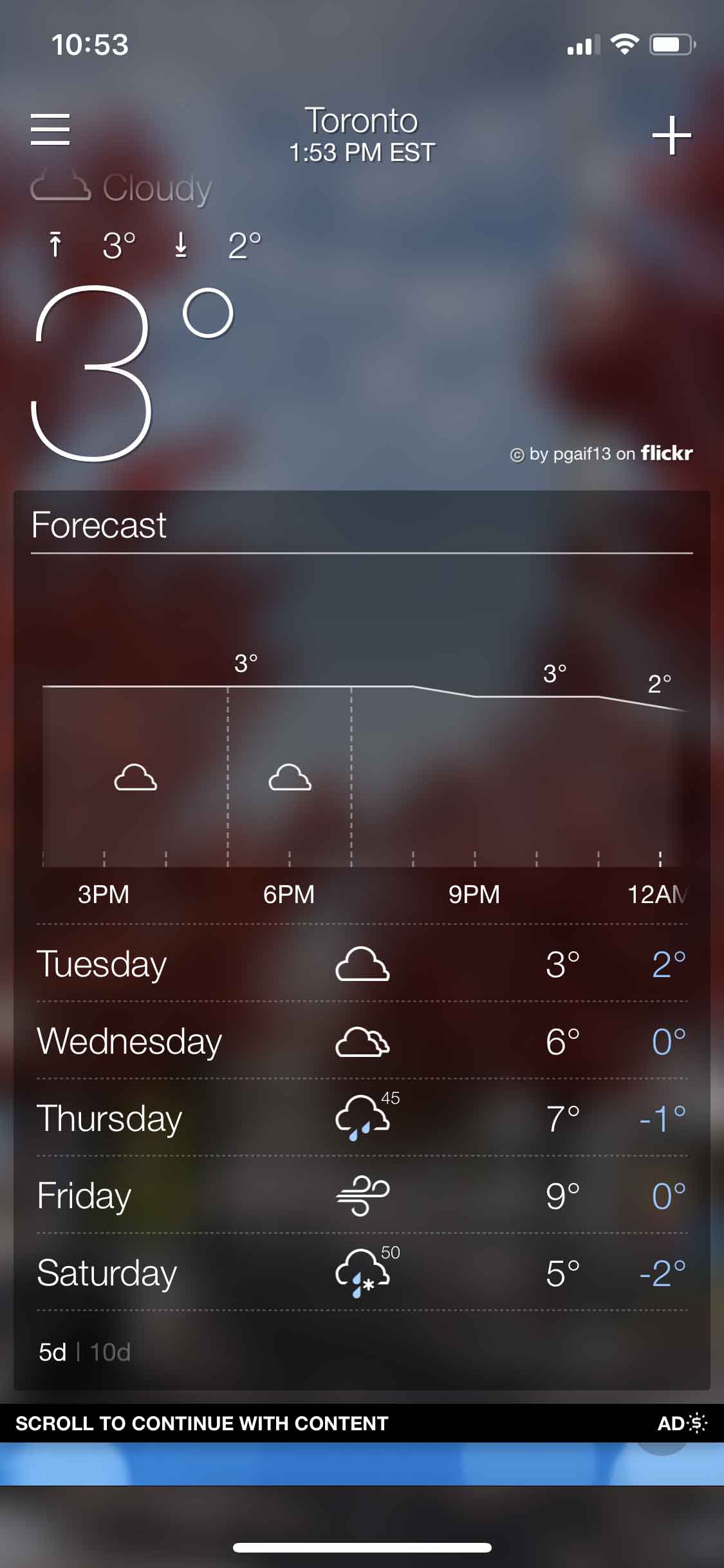This detailed caption accompanies a screenshot of a smartphone displaying a weather application interface. 

The background is gray and blurry, providing a neutral backdrop for the app's content. At the top of the screen, the status bar indicates it is 10:53 AM, with icons for network coverage, Wi-Fi, and battery life. Just below, the app specifies the location as Toronto and the current time as 1:53 PM EST.

The current weather is shown with a "Cloudy" label next to an icon of a cloud, accompanied by a temperature reading of 3°C. The day's high and low temperatures are 3°C and 2°C, respectively. The image includes a copyright notice by PGAIF13 on Flickr.

Further down, the app provides a 5-day weather forecast:
- Tuesday: Cloudy with a high of 3°C and a low of 2°C.
- Wednesday: Cloudy with a high of 6°C and a low of 0°C.
- Thursday: 45% chance of rain, depicted with a cloud and raindrop icon, with temperatures ranging from a high of 7°C to a low of -1°C.
- Friday: Windy conditions expected, with a high of 9°C and a low of 0°C.
- Saturday: 50% chance of rain and snow with temperatures varying from a high of 5°C to a low of -2°C.

Below the 5-day forecast, there is an option to extend the view to a 10-day forecast, which has not been selected. The screen prompts the user to scroll down for more content. At the bottom, there's a prominently displayed "ADD" button in white capital letters next to a white dollar sign.

The image is portrait-oriented, taller than it is wide, and notably devoid of people or animals.